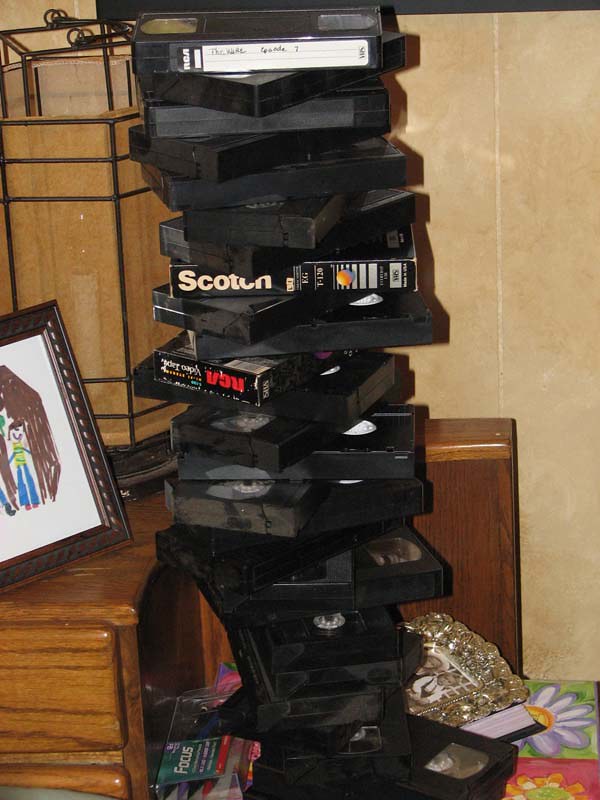This photograph, taken in someone's living room, captures a vertically stacked tower of black VHS cassette tapes, reminiscent of a Jenga tower with each tape slightly askew. Some tapes display the familiar white plastic centers and hand-labeled side labels, including one marked "Scotch." The scene features various background details; to the left, there's a partially visible medium-colored wooden nightstand. On the wall, you see a mix of art: a framed child's drawing depicting a person in blue jeans under a brown structure, a daisy illustration, and a gold ornate picture frame with a floral painting containing people. The setting includes brown cabinets, and the walls exude a peachy-beige hue. The photograph emphasizes the nostalgic VHS tower amidst a cozy, lived-in environment.